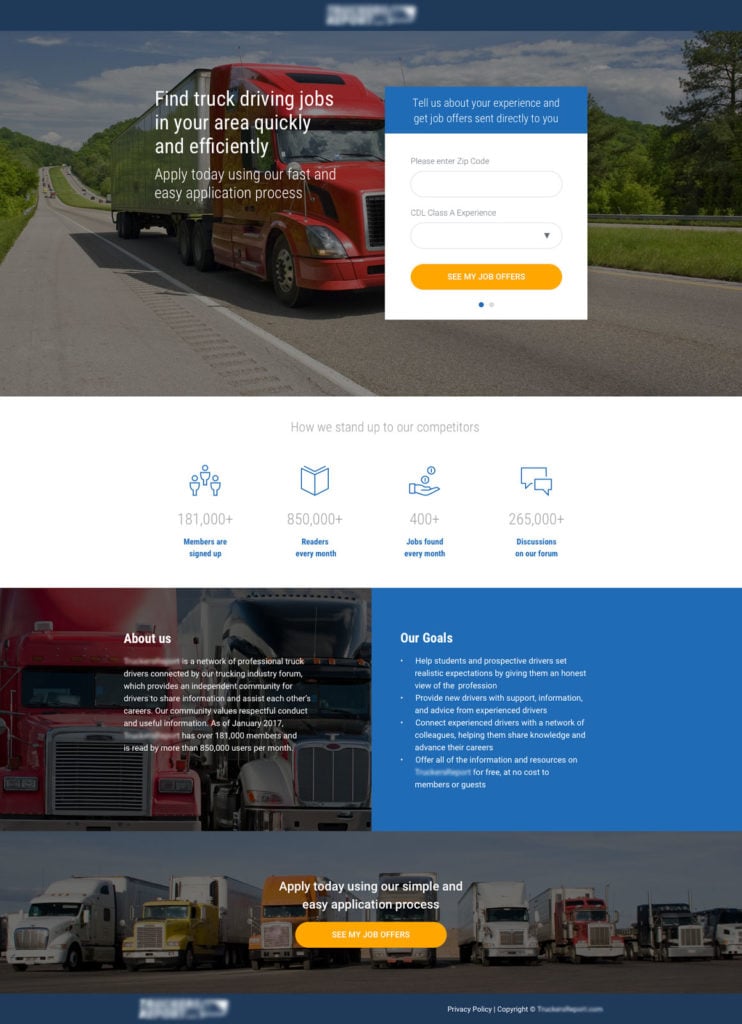The image consists of two screenshots, one positioned at the top and the other at the bottom, each showcasing various elements for a job application platform focused on truck driving opportunities. 

In the top screenshot, positioned against a scenic background of a rolling hills road flanked by lush trees, a red cab truck with a silver trailer is prominently featured. Overlaid at the center-left of the image is a message in white text that reads, "Find truck driving jobs in your area quickly and efficiently." Directly beneath this statement is a call to action: "Apply today using our fast and easy application process." A partially visible selection box with an orange button at the bottom is also present, though the contents within the box remain unreadable.

The middle portion of the top screenshot features four distinct icons arranged side by side. The first icon depicts three people, the second icon shows a book, the third icon illustrates a hand with coins falling out, and the fourth icon features conversation balloons. Underneath these icons, there is text in blue that is not legible. Additionally, below this section, another line of text reads: "About Us, Our Goals, and Apply today using our simple and easy application process," accompanied by an orange bar containing further unreadable text. The "About Us" section includes a paragraph, and the "Our Goals" section lists approximately six bullet points, both of which are too blurry to decipher.

The bottom screenshot showcases a row of eight tractor trailers aligned with their front noses pointing outward. This arrangement underscores the platform's focus on truck driving opportunities.

Overall, the screenshots emphasize the ease and efficiency of applying for truck driving jobs through a visually appealing interface, despite some illegible text components.